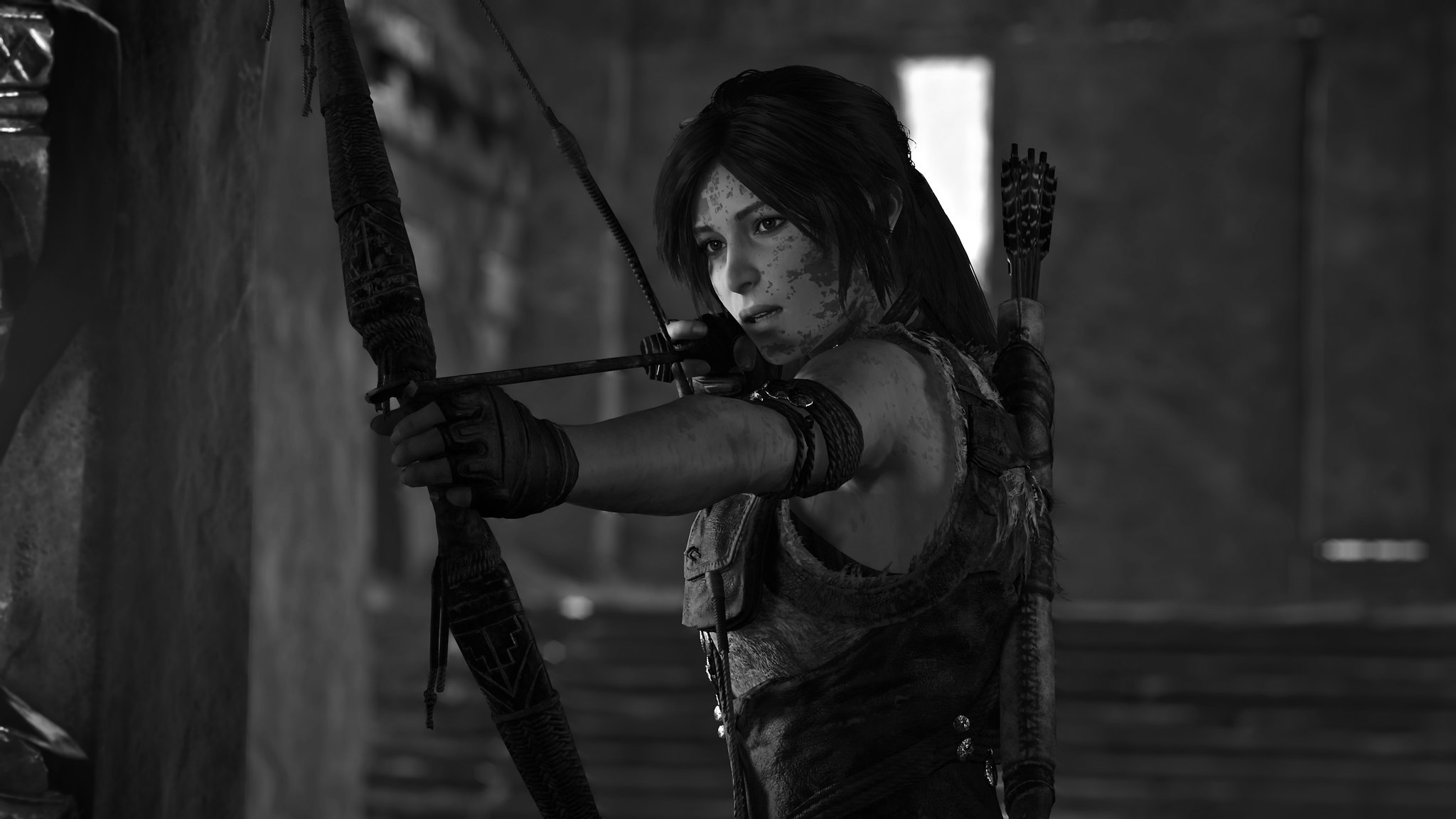In this striking black and white image, a scene reminiscent of a classic film or television show unfolds within what appears to be the rustic confines of a wooden shed or perhaps a stone building. The murky background subtly reveals a rectangular window, casting just enough light to highlight the central figure dominating the composition. At the heart of the frame, a woman stands poised and resolute, captured in profile as she readies to release an arrow from her imposing bow. 

Her posture is diagonal, with her left forearm and shoulder prominently facing the camera, pointing leftward, while her right elbow is drawn back, poised in the top right corner, signaling her imminent shot. Her long black hair cascades down, creating a stark contrast against her intense, focused expression locked onto her target. Leather straps encircle her left upper forearm, hinting at her combat proficiency, while a tactical vest snugly fits her torso. On her back, a quiver with a couple of arrows indicates her readiness for action. The large bow she wields, although resembling a crossbow at the front, is distinctly not one, adding to the intrigue of her gear. This evocative image brilliantly captures a moment of concentration and skill in a beautifully composed scene.